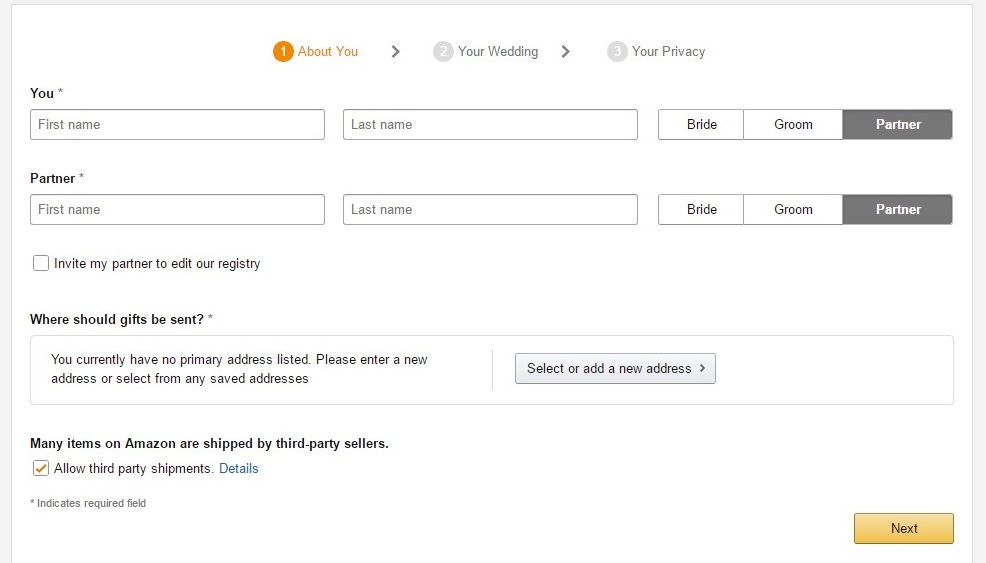The image appears to be an Amazon sign-in interface, divided into several distinct sections. At the top center, there are three categories marked by numbered circles and labeled text. 

1. The first category, labeled "1. About You," features white text on an orange circular background and has an arrow pointing to the right. 
2. The second category, labeled "2. Your Wedding," is grayed out. It has a white number 2 in a gray circle, also with a right-pointing arrow beside it. 
3. The third category, labeled "3. Your Privacy," similarly features a white number 3 in a gray circle and is grayed out.

In the middle section, starting from the far left, the word "You" is displayed with a box below labeled "First Name." Adjacent to this, there is another box labeled "Last Name." To the right of these, three vertically separated boxes are labeled "Bride," "Groom," and "Partner."

Further below, under the section labeled "Partner," there are similar fields: "First Name," "Last Name," and the options "Bride," "Groom," and "Partner."

On the bottom left of the interface, there is a note stating, "Many items on Amazon are shipped by third-party sellers." Below this, there is an option to "Allow third-party shipments," accompanied by a box with a question mark inside it.